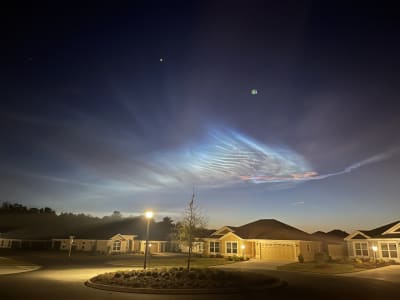This detailed photograph captures a serene suburban neighborhood at night. In the foreground, there's a roundabout featuring a central island adorned with a tree and small bushes. Nearby, a lamppost illuminates the scene. Surrounding the roundabout are single-story houses with lit driveways, garage doors, and illuminated windows, all contributing to a tranquil atmosphere. The image extends into the background where the silhouettes of trees and a dense woodland are faintly visible under the night sky. The sky itself is a striking focal point, showcasing an array of lit clouds with a sunset blending into the oncoming night, a unique angel-like cloud formation emitting a soft white glow, and two visible stars - one notably larger than the other - in the upper center of the scene. The overall composition evokes a homely, peaceful night in the suburbs.